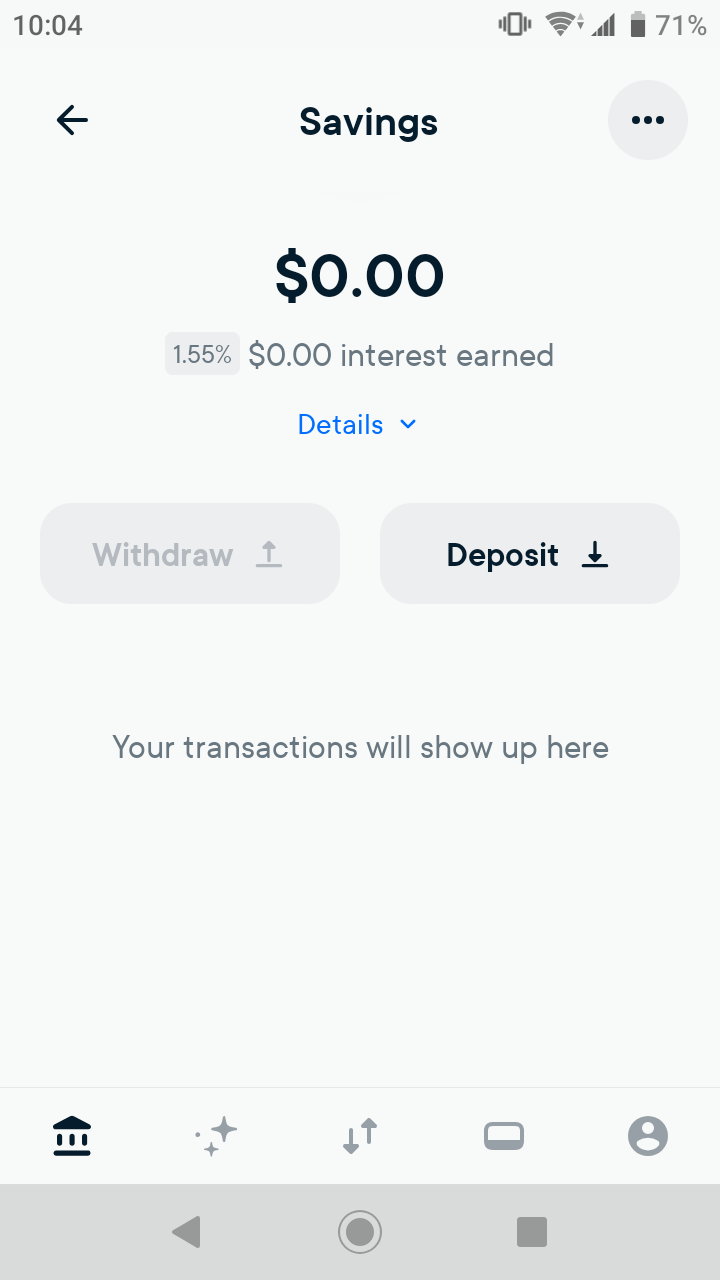The image displays a smartphone screen with various UI elements and status indicators. 

In the upper left corner, the time is shown as "10:40," while the upper right corner displays "10:04," suggesting a minor discrepancy. Below the time, the status bar indicates the phone is on vibrate mode, with Wi-Fi and cellular data icons, signal strength bars, and a battery level of 71%.

Directly below the status bar, there is a navigation section with a left-facing arrow labeled "Savings" on the left, and a circular icon with three vertically arranged dots on the right.

The primary interface below this section shows account information. It features:
- A balance of "0.00"
- An interest rate of "1.55%"
- An interest earned of "0.00"

Additional information is accessible via a blue-highlighted "Details" dropdown. Below this, two buttons are present: a gray "Withdrawal" button with gray text, and a "Deposit" button, which is gray with black text. There are no transactions listed, as indicated by the text, "Your transactions will show up here."

The lower portion of the screen features a horizontal white band with several icons:
- A building resembling a bank
- Three four-pointed stars
- Upwards arrows and a single downward arrow
- A card icon
- A profile icon depicting a circle with a person inside

At the very bottom is a navigation strip colored in gray, which includes a left-facing arrow within a circle on the left, and a square icon on the right.

The screen's color palette consists primarily of white, gray, black, and blue. The display format is longer vertically than horizontally, making it noticeable in size yet not requiring magnification for clarity.